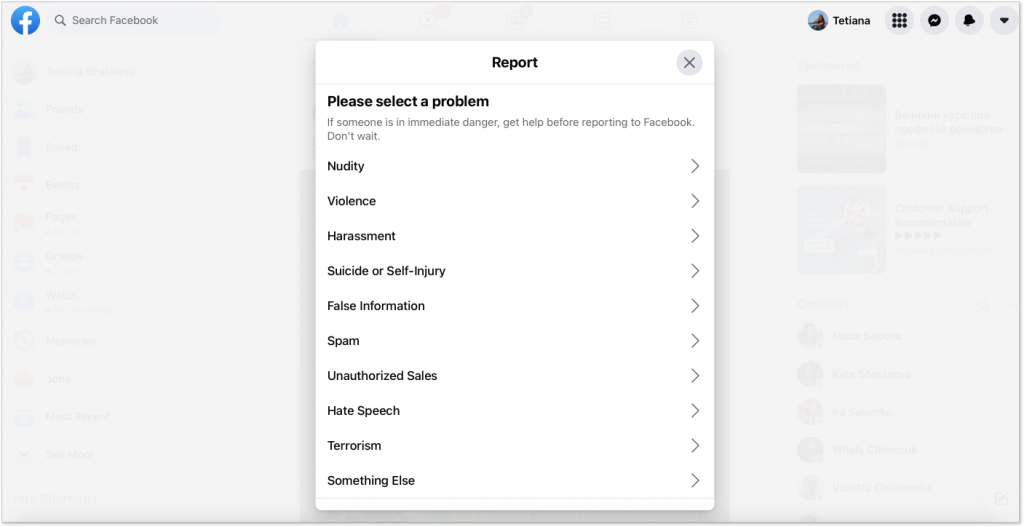The image captures a user interacting with Facebook's search feature. The screen displays grayed-out menus and search results to the left and right, emphasizing the active window. At the top, the Facebook header is visible, featuring the 'Tetiana' logo alongside a grid of icons for chat, notifications, and reactions.

Dominating the center of the screen is a prominent report panel with a heavy drop shadow effect, drawing the viewer's attention. The panel's header reads, "Please select a problem," followed by a critical advisory: "If someone is in immediate danger, get help before reporting to Facebook. Don’t wait."

Below this message, a list of reportable issues is presented in black text with thin gray arrow buttons to the right of each option. The issues are listed vertically and include:
- Nudity
- Violence
- Harassment
- Suicide or self-injury
- False information
- Spam
- Unauthorized sales
- Hate speech
- Terrorism
- Something else

Each category is designed to help users identify and report a wide range of problems that may occur on the platform.

The rest of the screen remains grayed out with a semi-transparent white overlay, highlighting the report panel as the focal point. Once the reporting process is completed, the user interface is expected to return to the standard website view.